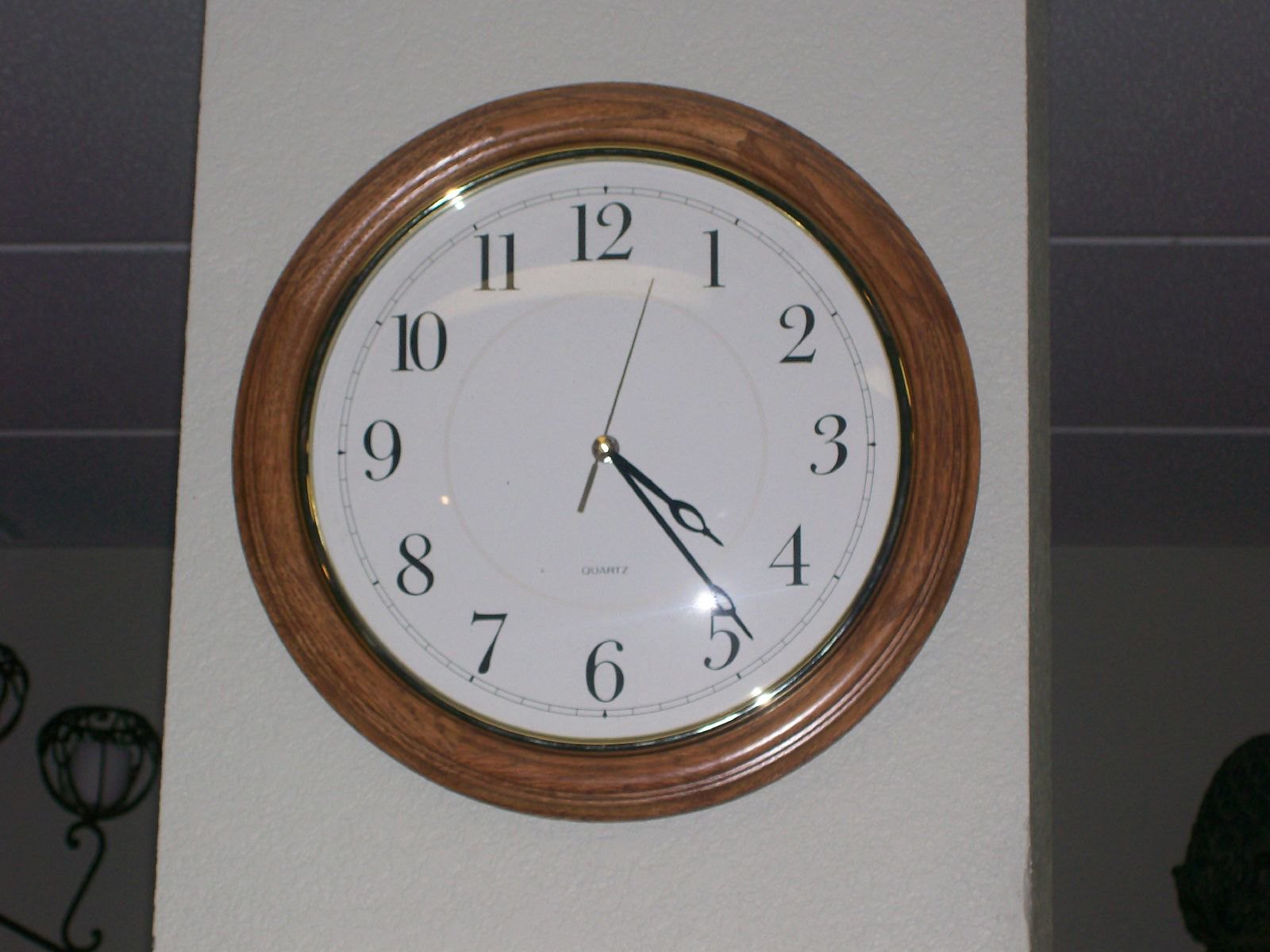This color photograph features a central segment of a whitish-gray wall. Dominating the wall is a round clock with a wooden rim, encircling a thin, gold-colored inner rim that borders the clock face. The face of the clock is white, accented by a small border just beyond the start of the white area. The numbers on the dial are rendered in black, and the clock features three hands: a minute hand, an hour hand, and a gold second hand, which is pointing to approximately 3 seconds. The time displayed is 4:24. Above the wall, the ceiling is visible, comprised of patterned tiles. In the left-hand corner of the photograph, there is a black wrought iron ornamentation, possibly a decorative plaque.